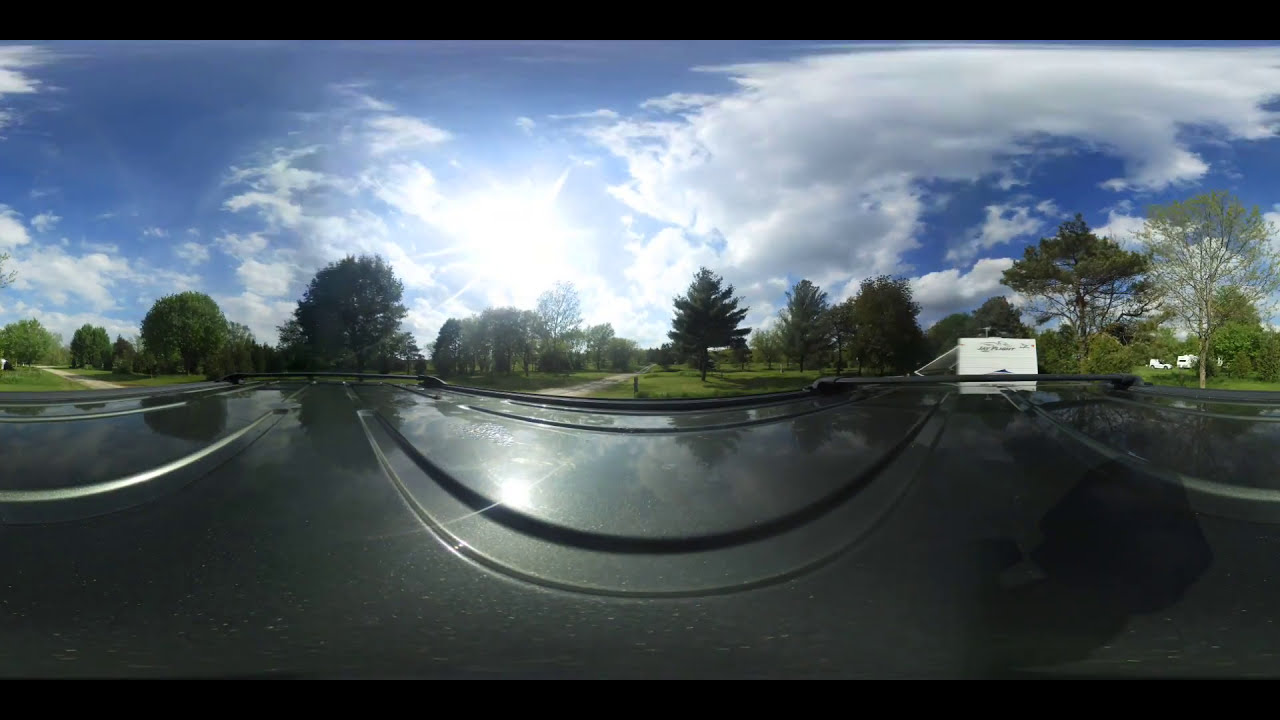The image appears to be a panoramic shot, likely taken from a car, which has resulted in some distortion. The foreground is dominated by the view of the car’s dashboard or hood, creating a shiny, metal-like surface that distorts into the scene. In the midground and background, a park-like area unfolds, characterized by lush greenery with numerous trees and grassy patches. There are a couple of paths visible, though the distortion makes it hard to tell if there's more than one. The photo captures a motorhome on the far right and a truck slightly to the left of it, with a white sign even further to the left. Above, the sky is vividly blue, scattered with sizable clouds, and the sunlight makes the scene appear bright. Despite the warping of the image, the composition suggests a serene outdoor environment possibly near a roadway or an open area frequented by vehicles.